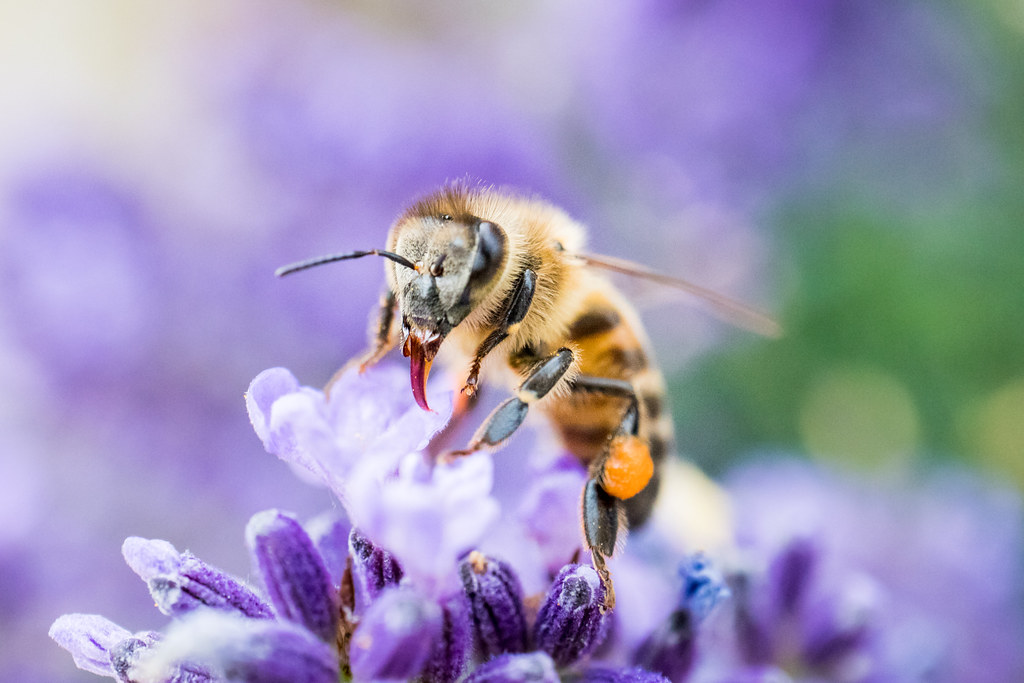A detailed photograph captures a bumblebee poised on a vibrant purple flower, collecting pollen. The bee, marked by its distinctive yellow and black body, is positioned diagonally with its head facing the left and its body towards the right. Its antennae are clearly visible, and a prominent black horn-like structure protrudes from the center of its forehead. The bee appears to be extending a purple tongue-like appendage towards the flower, possibly to gather nectar. Its eye is egg-shaped, and the yellow ball of pollen clinging to its second or third leg on the left side adds to the detail. The bee's translucent wings with dark edges stand out against the multiple bright purple sections of the flower. Additional purple flowers can be observed in the background, enhancing the overall vividness of the scene.